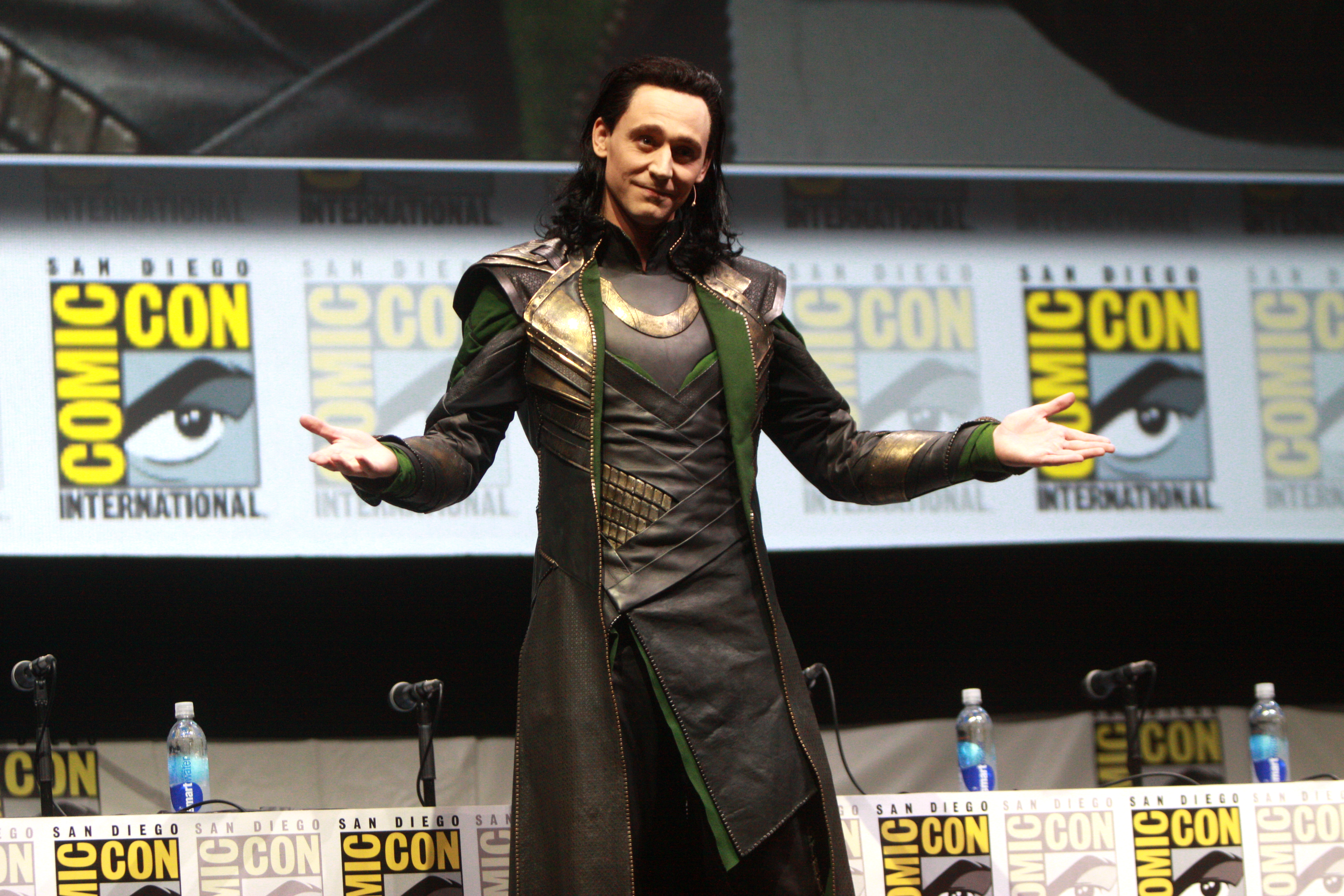This image is a detailed photograph of the actor who portrays Loki in the Avengers movies, captured at Comic-Con International in San Diego. He stands prominently in the center, fully donned in his intricate olive green and brown leather costume, highlighted with gold accents around the neck, sleeves, and shoulders. His hair, shoulder-length and black, frames his face as he gazes forward with his head slightly cocked to the right, creating an engaging and dynamic expression. His arms are extended outward, palms facing up, in a signature Loki pose.

In front of him stretches a long table adorned with Comic-Con posters, black microphones, and several small plastic bottles labeled "smartwater." The backdrop behind the table consists of a black wall featuring a large horizontal banner filled with Comic-Con logos. Above this banner, the background transitions from dark on the left to white on the right, creating a contrasting visual effect. The entire setup situates him within the energetic and bustling atmosphere of Comic-Con, emphasizing the significance of the event.